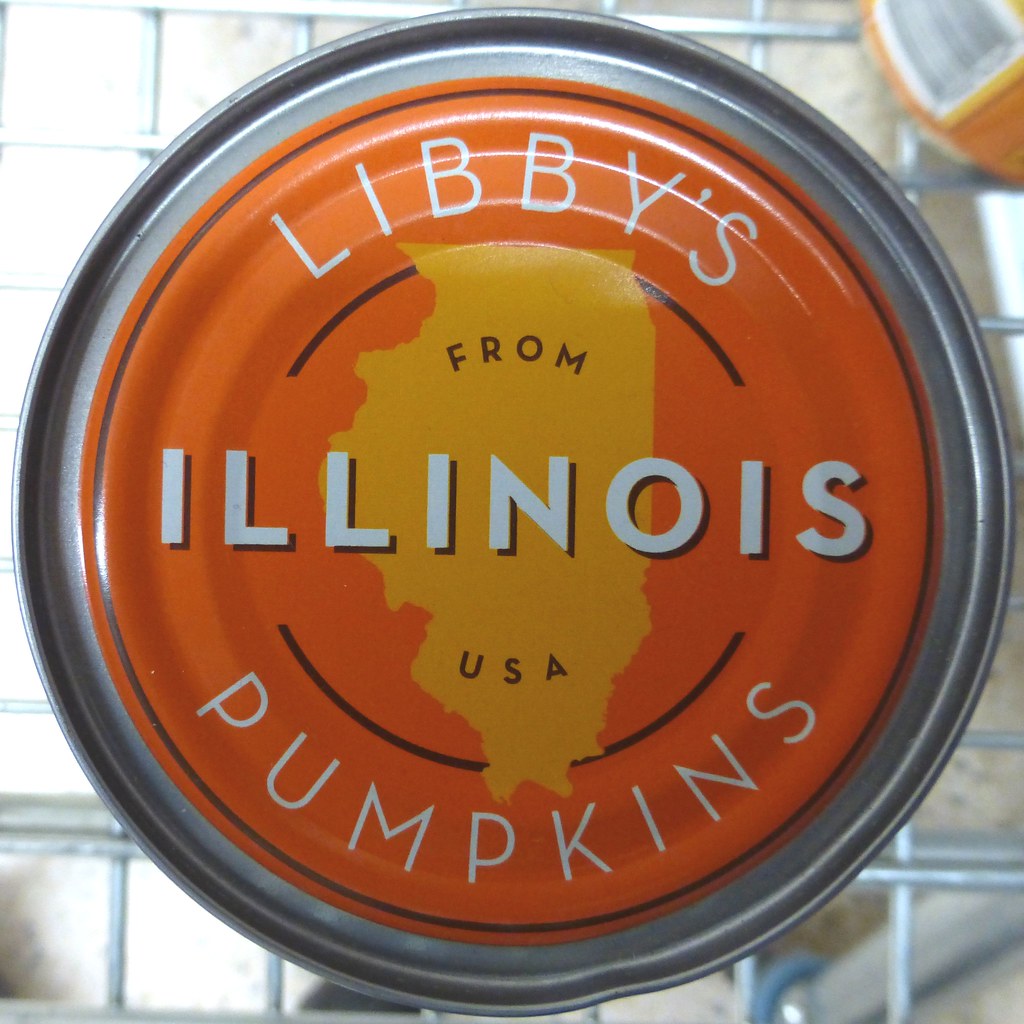This is a full-color photograph showcasing the top view of a slightly dented can, prominently featuring the label. The outer rim of the can is silver, while the top surface is painted orange. In the center, a yellow silhouette of the state of Illinois is displayed. Surrounding the silhouette, the text "Libby's" is curved at the top in white letters with ample spacing, accompanied by a dark gray shadow. Below it, in a straight line, "Illinois" is written in white with a gray drop shadow. Curved like a smile at the bottom, the word "Pumpkins" is also in white. At the top of the Illinois silhouette, "from" is written in gray, and at the bottom, "USA" can be seen. Behind the can, a metallic grill suggests it may be inside a shopping cart, with the bars visible underneath and possibly another can nearby.